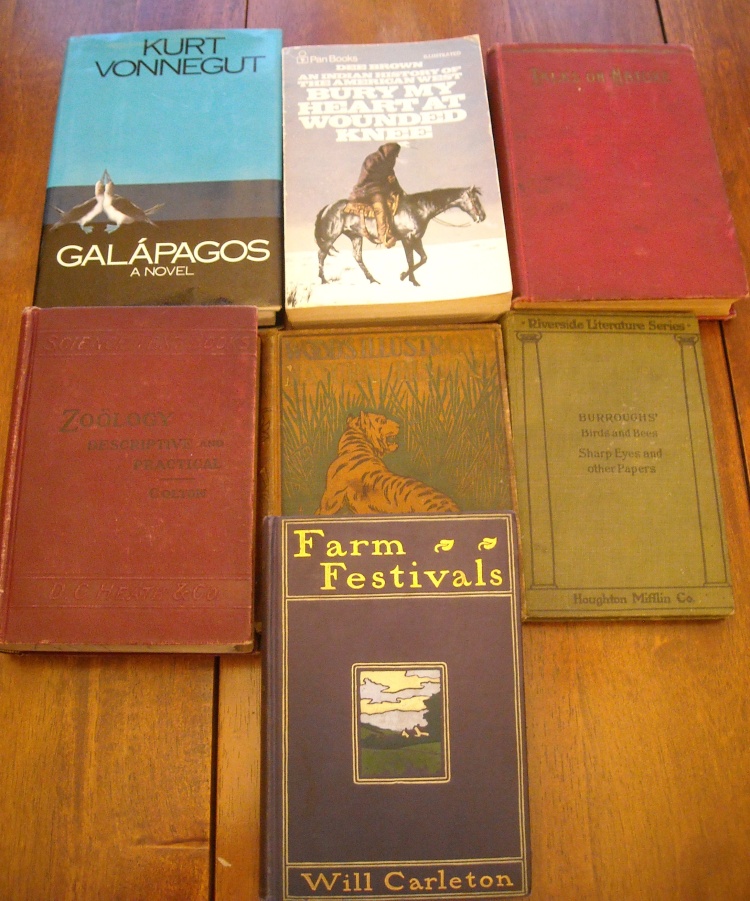This image showcases seven books laid out neatly on a varnished wooden table with visible sections between the planks. The top row includes three books: the first has a blue and black cover titled "Galapagos: A Novel" by Kurt Vonnegut; the middle one is "Bury My Heart at Wounded Knee" featuring a white background with an illustration of a man riding a horse; the third book on the top row has a faded red cover, making the title difficult to discern. The second row also contains three books: the leftmost has a red cover and is titled "Zoology, Descriptive and Practical" by Colton; the center book has a green and yellow cover with an image of a tiger in the grass, but the title is hard to make out; the book on the right side of the second row is green and titled "Burroughs, Birds and Bees: Sharp Eyes and Other Papers," published by Houghton Mifflin Company. At the bottom, lying partially on top of the center book with the tiger, is a burgundy book titled "Farm Festivals" by Will Carlton, featuring a small illustration of a field and sky on its cover.